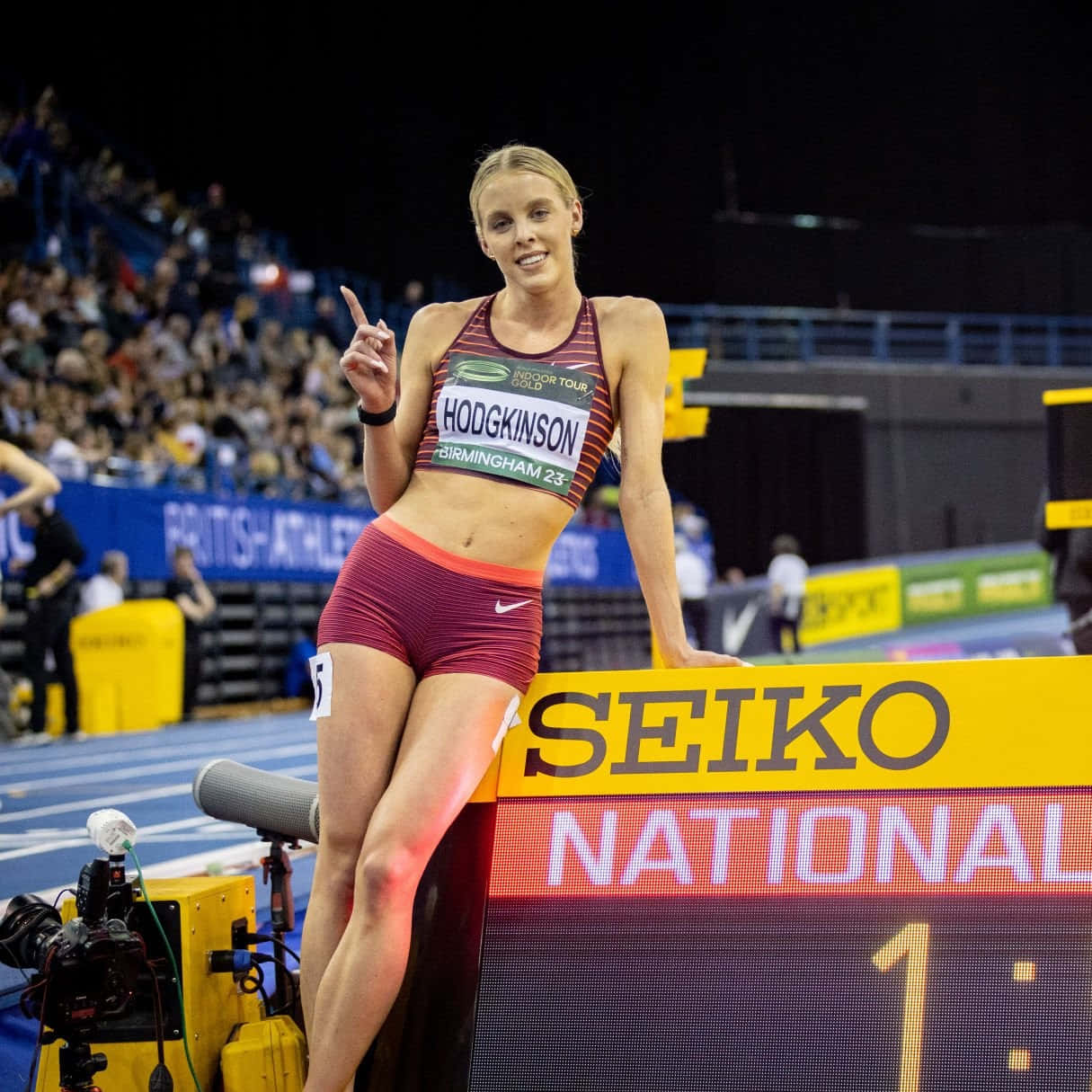The image captures a victorious female athlete named Hodgkinson in a stadium during the Seiko National Indoor Tour Gold event, identified as Birmingham 2023. She is dressed in a Nike track outfit consisting of red athletic pants and a red and tan vertical striped tank halter top, adorned with stickers displaying her race number five on the outsides of her thighs. Prominently displayed on her top is a large badge reading "Indoor Tour Gold Hodgkinson Birmingham 23." Hodgkinson, a blonde, looks incredibly fit and is captured alongside recording equipment assumed to be for tracking photo finishes. She proudly leans against a board emblazoned with "No. 1," sponsored by Seiko, raising her right index finger to signify her first-place win. The background reveals a crowd-filled stadium with blue banners proclaiming "British Athletics," underscoring her affiliation and triumph in the event.